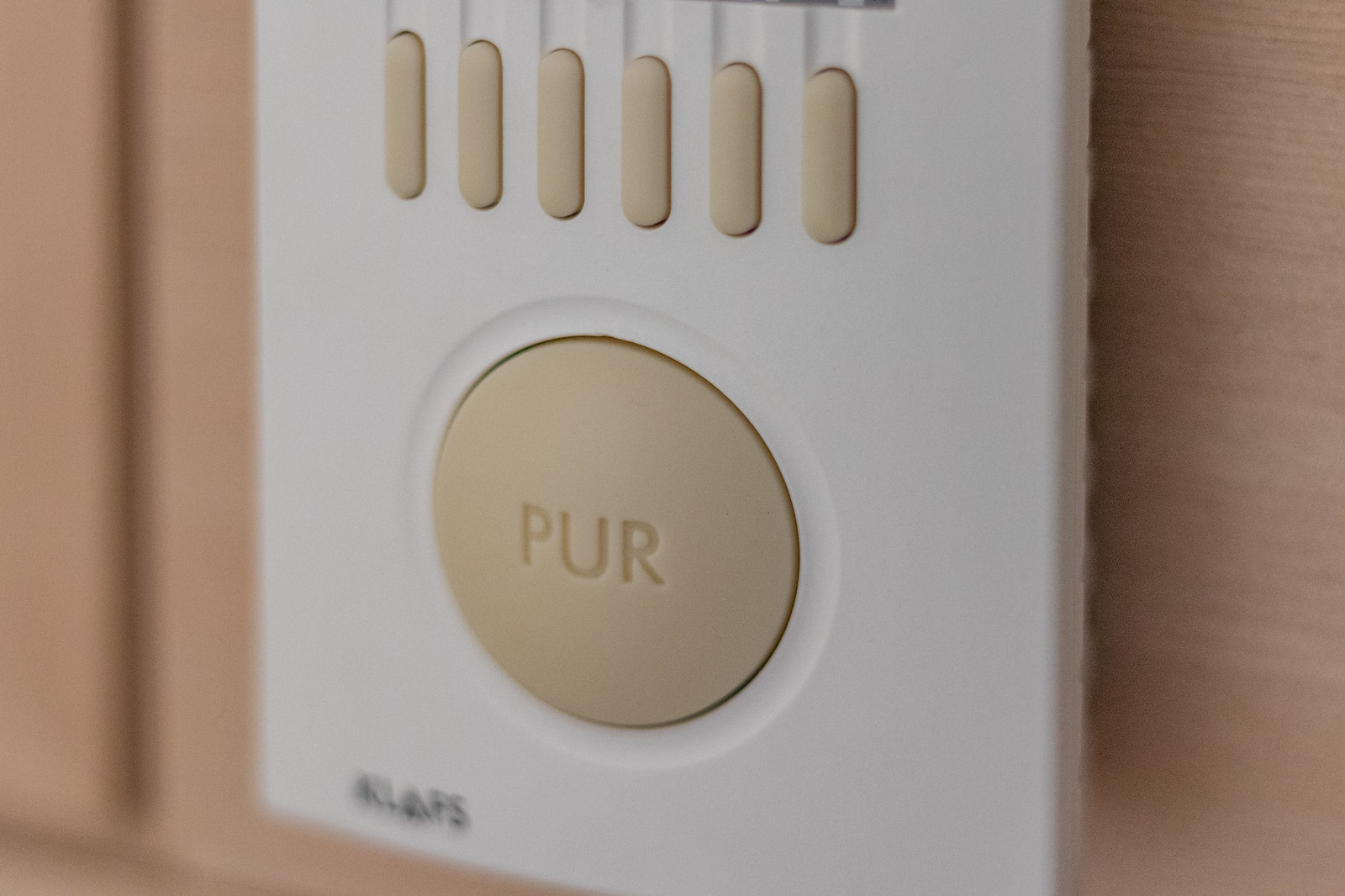This image features a close-up shot of a mounted device. The focal point is a rectangular white device, of which only the bottom portion is visible. Positioned centrally on this section is a large, round, beige button inscribed with the capital letters "P," "U," and "R." Just above this, a horizontal line of six small, pill-shaped beige buttons is set into grooves matching their shape. In the bottom left corner, the somewhat blurred and faded text appears to spell "K-L-A-P-S," though this is not entirely clear. The device is attached to a wall or surface resembling a sandy beige color, echoing the hue of the buttons but with a more reddish undertone. The background is blurred but includes a noticeable line on the left side, suggesting a cabinet or some form of separation in the wall.